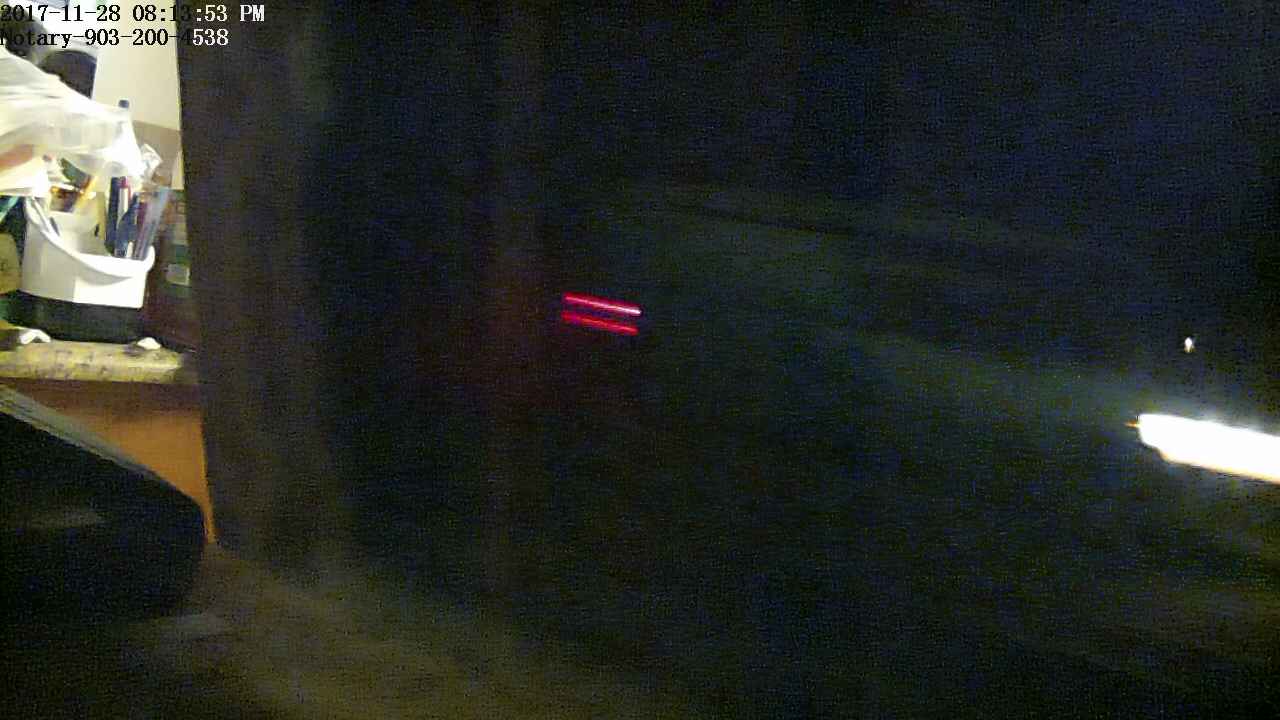This color photograph, taken at night, is dark, blurry, and grainy, making it challenging to discern specific details. Toward the upper left-hand corner, there is some text in black and white, possibly including a date and a series of numbers, though it is difficult to read. In the left-hand corner, an illuminated window, possibly belonging to a shop or store, is visible. Inside, a white object holds what might be blue bottles or glasses, and there is possibly a person in a white jacket with a black rim at the bottom, appearing to stir a pot. This scene rests upon what seems to be a granite or wooden shelf. A large window or door occupies most of the picture, revealing the outline of a vehicle beyond it. The vehicle's front lights appear toward the right edge, accompanied by a small light above them. Reddish backlights are visible near the center of the image.